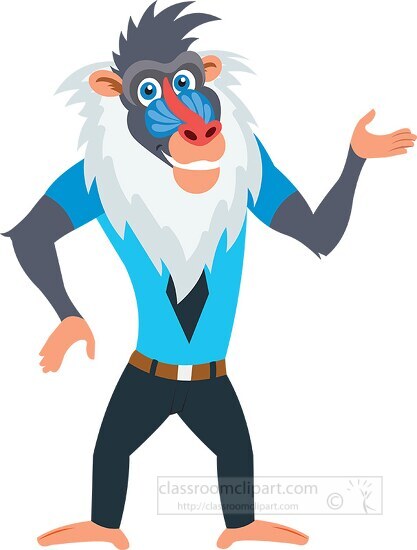This image depicts a striking, colorful cartoon character resembling a half-gorilla, half-baboon hybrid with a whimsical and fun appearance. The character stands upright, barefoot, with arms extended, exuding a lively and animated vibe. He has a distinctive baboon face characterized by vibrant red and blue hues, a large gray mane like fur around his face, and expressive big blue eyes. His outfit consists of a long-sleeve gray shirt beneath a Carolina blue short-sleeve T-shirt adorned with a black diamond on the front. Completing his attire are navy blue pants cinched with a brown belt featuring a white square buckle. His hair stands up like a mohawk, adding to his playful and dynamic look. There is a watermark at the bottom right corner that reads "classroomclipart.com," indicating it is a digital clipart image. The character's fun yet gentle appearance, highlighted by a comical red nose and a bright smile, makes the overall drawing visually appealing and very colorful.